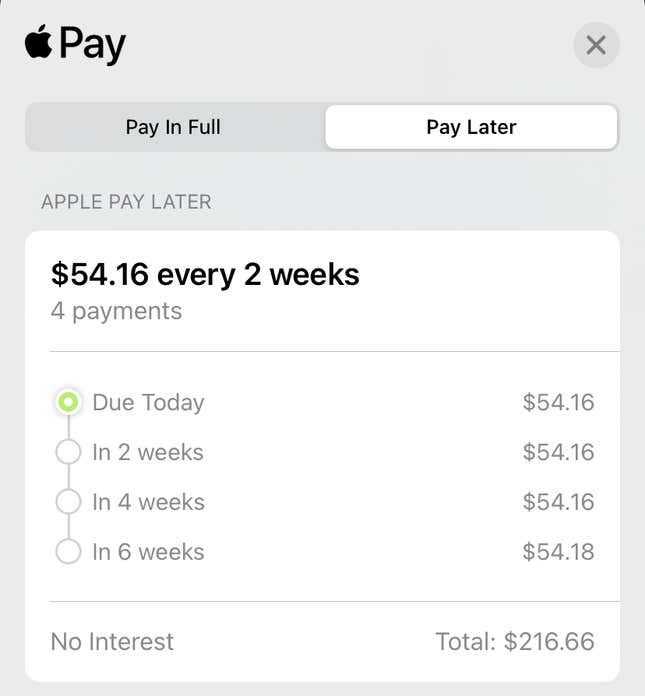This image features an Apple Pay Later receipt against a gray background. Prominently in the upper-left corner is the Apple Pay logo, which consists of an apple with a bite taken out of the right side, followed by the word "Pay" in black text. On the upper right side of the image is a large "X".

Central to the image is a large white square located at the bottom middle. Inside this square, at the top, are two payment options: "Pay in Full" and "Pay Later," with "Pay Later" highlighted in white. Below these options, within the white square, is a detailed breakdown of the Apple Pay Later plan. 

The plan specifies that payments of $54.16 are to be made every two weeks. It details four segmented payments, each labeled respectively as "Due Today," "In Two Weeks," "In Four Weeks," and "In Six Weeks." Each payment is $54.16, except for the final payment in six weeks, which is slightly higher at $54.18.

At the bottom of the white block, a dividing line separates additional information. On the bottom left, it states "No Interest," while the bottom right mentions "Total: $216.66." 

All written content within the white square is in gray text, with the exception of "$54.16 every two weeks," which is in bold black font for emphasis.